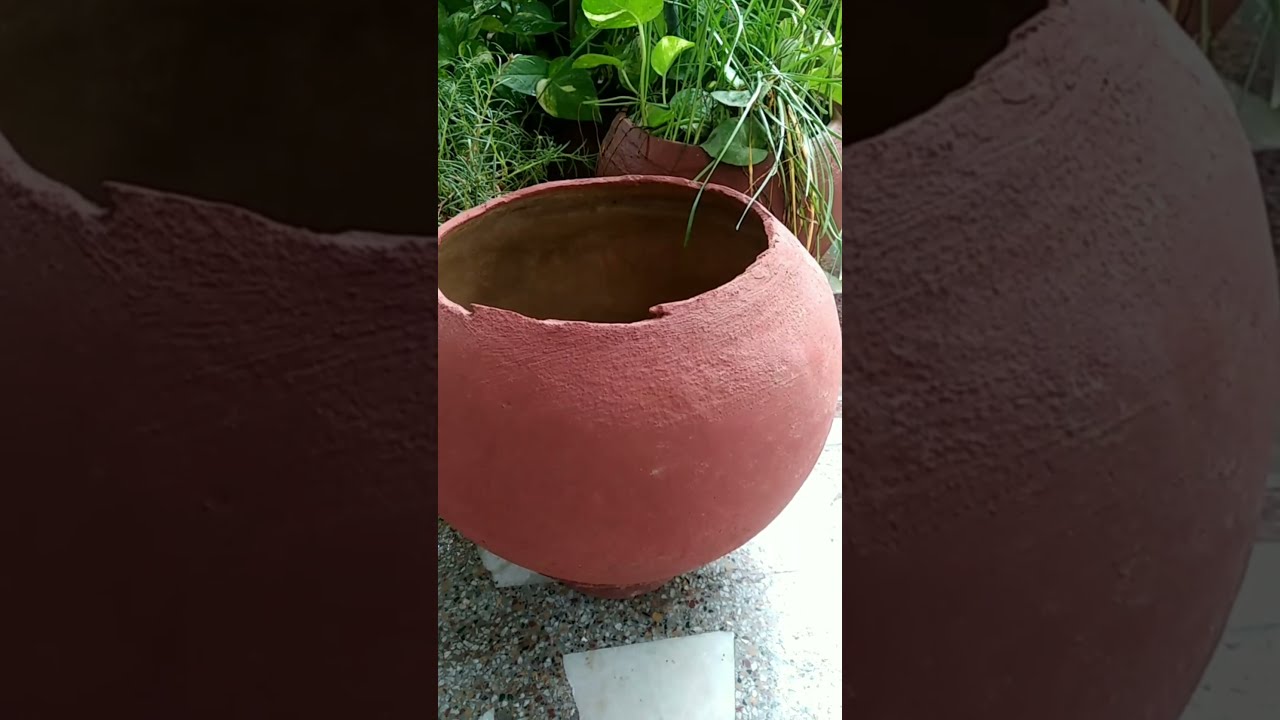This three-panel image features an outdoor setting, with the central panel brightly illuminated by natural sunlight, contrasting with the darker side panels. The centerpiece of the composition is a distinct stone wall, encrusted with pebbles and partially bathed in natural light from the right. In front of this wall sits a distinct reddish-brown clay pot, characterized by its irregular and jagged upper rim. The pot is empty and has a textured surface, especially noticeable around its upper edge. Behind this pot, a similar pot in color and texture holds a variety of green plants. These plants range from long, thin grass-like strands to fuller leaves that resemble nasturtium, pothos, or possibly peperomia. Additionally, sprigs of rosemary or tarragon can be seen around and behind the potted plant. The base of the pots rests on a platform of dark gray concrete with white gravel highlights, adding to the image's intricate details and depth. On the left side of the panel, there is a patch of green grass, adding a natural frame to the outdoor scene.